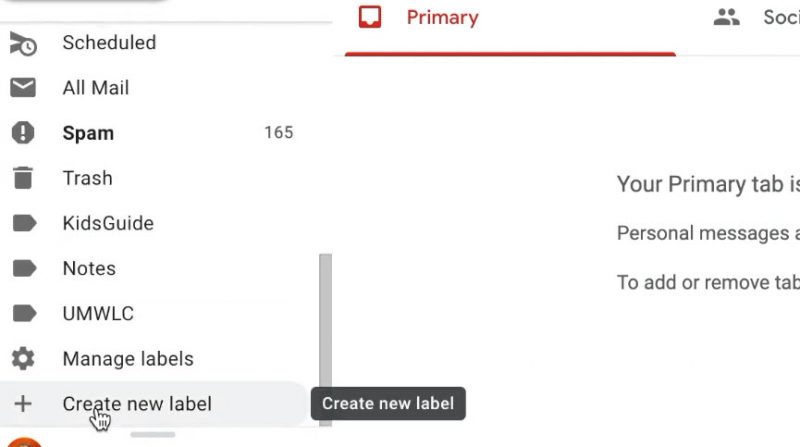This detailed screenshot from Google Mail showcases the interface with various sections visible on the right side of the screen. These sections are organized vertically and include tabs for "Scheduled," "All Mail," "Spam," "Trash," as well as several user-created labels such as "Kids Guide," "Notes," "UMWLC," and "Managed Labels." At the very bottom of this list is an option labeled "Create New Label," which appears highlighted in a slightly darker gray, indicating it is currently selected by the user. 

To the left, a text box appears with the black words "Create New Label," signifying the user's action of initiating the creation of a new label. Above this, the "Primary" tab is prominently highlighted in red. A partially visible message reads "Your primary tab," with some words obscured, and suggests instructions or information related to managing the primary tab and its messages.